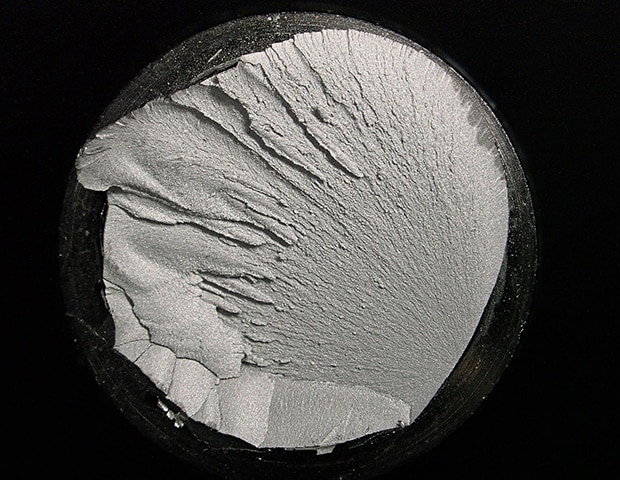The image showcases a round, cylindrical object set against a completely black background. The exterior of the object is covered in a textured black surface, resembling tiny sand particles. The object has been cut open cleanly, revealing an interior of light gray with an earthen, sand-like texture interspersed with ridges and folds. The interior surface transitions from rough and overlapping textures at the top left to smoother areas towards the bottom. The overall appearance suggests a contrast between the dark, possibly wooden exterior and the lighter, intricately textured interior, emphasizing its inanimate, possibly artistic or natural origins.